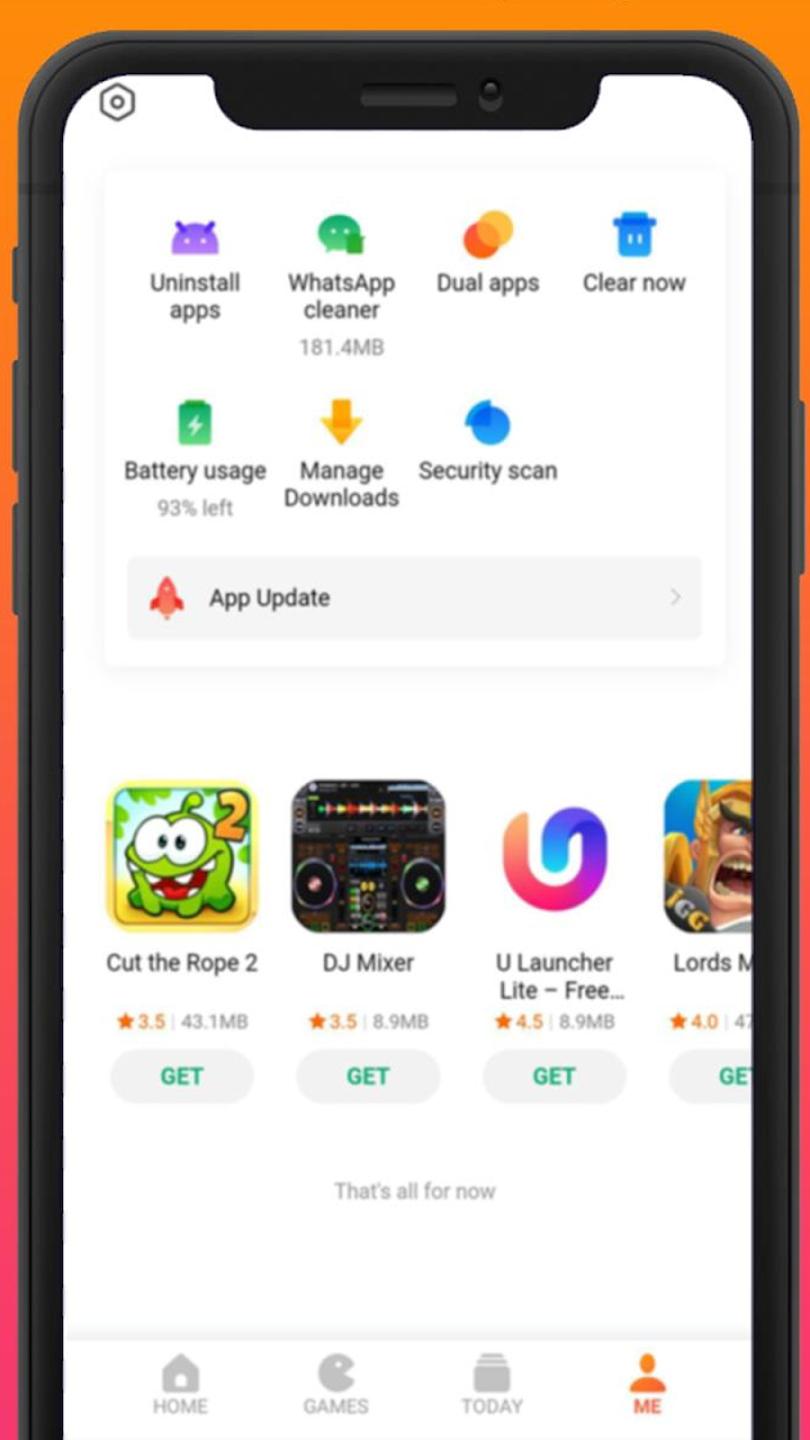The image is a detailed digital composition of a mobile phone screen, enclosed in a sleek black case, set against an orange and pink gradient background. At the top of the phone, both a camera and a microphone or speaker are evident, lending realism to the graphic. The home screen within displays an application, resembling an app store, showcasing various downloadable mobile applications. A navigation menu is prominently positioned at the bottom, featuring sections such as Home, Games, Today, and Me, with the 'Me' section highlighted in orange.

The upper portion of the screen showcases seven clickable icons for different utilities, including 'Uninstall Apps', 'WhatsApp Cleaner', 'Security Scan', and 'Manage Downloads', among others, indicating various features or statuses. Below these options, advertisements appear, presenting icons of different apps available for download, each accompanied by a brief review, app size, and a prominently placed 'Get' button for easy access.